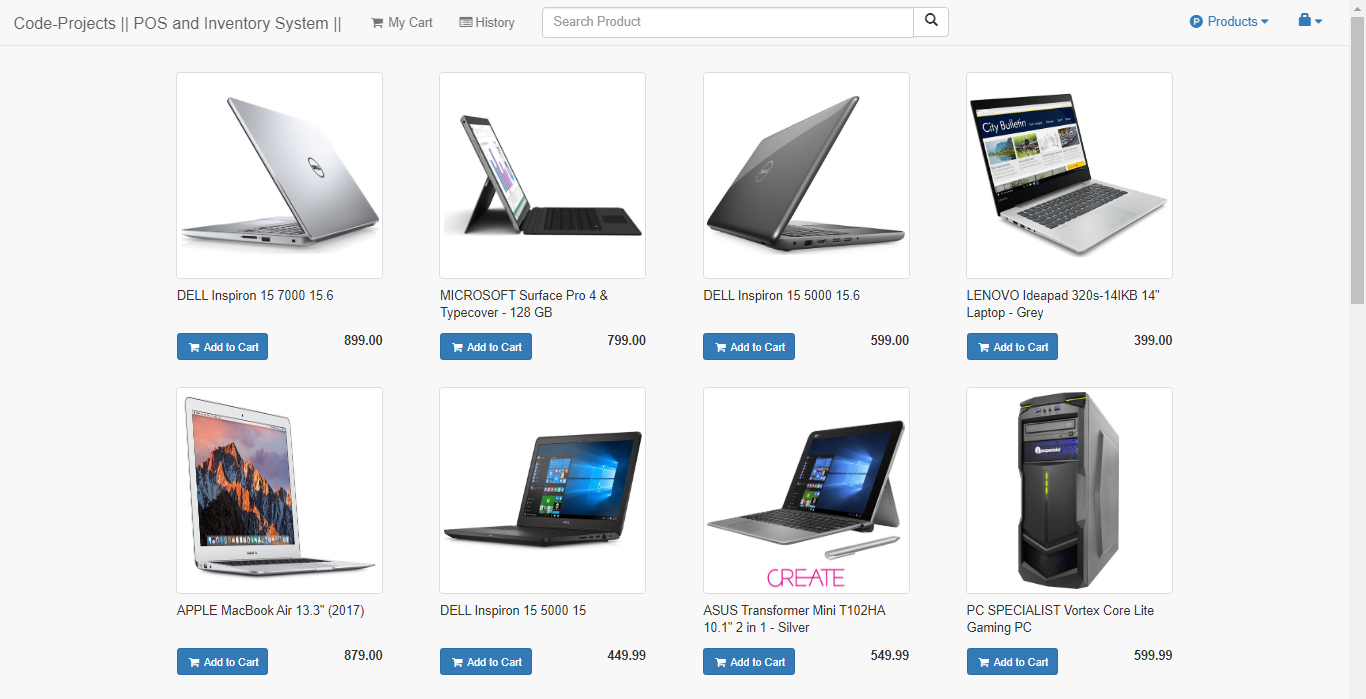The image showcases a user interface for "Code Project 2: POS and Inventory System." At the top, several navigation options are visible, including "My Cart," "History," and a search bar labeled "Search Product." A blue hyperlink labeled "Product" features a drop-down menu, as does an adjacent lock icon.

Below the navigation bar, there are eight distinct white squares, each displaying an image of a laptop or a similar computing device. Under each image, a blue "Add to Cart" button is positioned on the bottom left.

Details for the products are as follows:

- The product in the top left square is a "Dell Inspiron 157000, 15.6," priced at $899.
- Next, the "Microsoft Surface Pro 4 and Type Cover, 128 GB," is listed for $799.
- Below that, another "Dell Inspiron 155000, 15.6" laptop is priced at $599.
- The final product in the sequence is a "Lenovo IdeaPad 320S, 14 KB, 14 inch laptop, gray," available for $399.